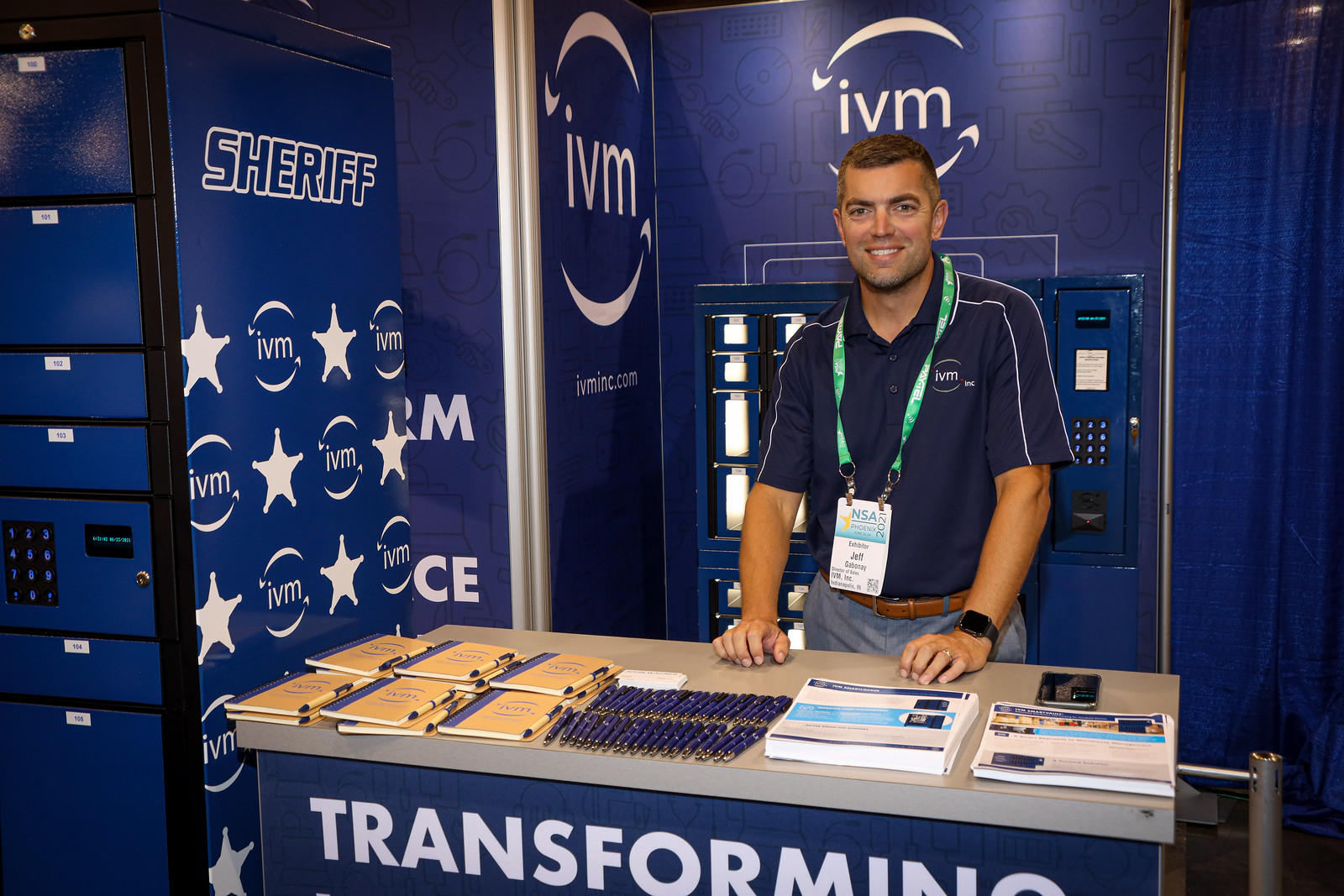The photograph depicts a representative standing behind a booth at a convention. He is dressed in a dark blue polo shirt with white piping and a logo on the chest that reads "IVM," framed by white arches. Around his neck, he wears a lanyard with a name tag, and he's also sporting a black smart watch. The booth's counter is organized with blue pens, notebooks, brochures, and flyers. The front of the counter features a blue banner with white letters saying "transforming." To his left, a blue panel displays the word "Sheriff" in white letters, interspersed with white stars and the IVM logo, which also appears behind him. An ATM machine is partially visible against the blue backdrop behind him. Near his shoulder, the URL "IVMINC.com" can be seen. The man is smiling for the camera, ready to interact with attendees.